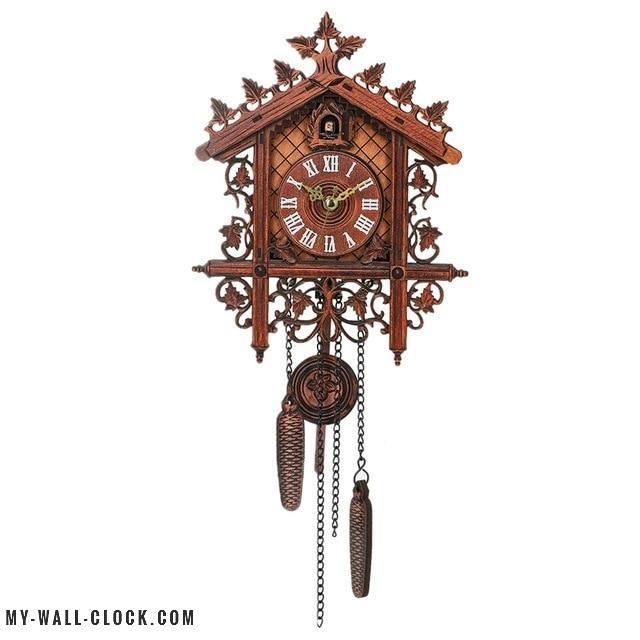The image features a brown wooden cuckoo clock intricately shaped like a house, enhanced with ornate leaf carvings around its perimeter. Set against a white background, the clock displays Roman numerals and is equipped with a brass hour hand, minute hand, and a thin second hand, currently showing the time as 10:09:33. At the bottom, four chains dangle from the clock, with two acorn-shaped counterweights attached to the middle chains, a disc in the center, and another pine cone weight lower on the right. A mechanical door pops open every hour to reveal a bird that makes a cuckoo sound. Additionally, there is a watermark on the bottom left of the photo that reads "my-wall-clock.com."